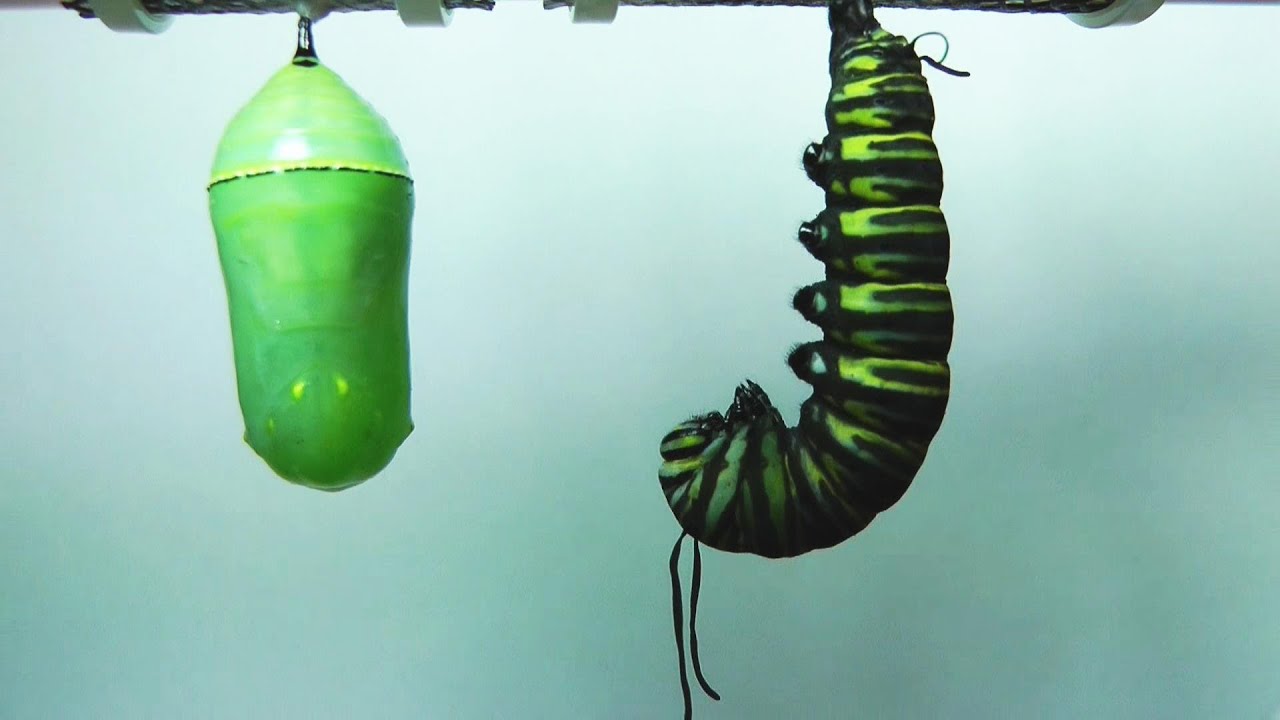In the image, a vibrant green and black striped caterpillar with two long antennae and smooth, hairless skin, hangs from its hind feet next to a green hummingbird feeder. This feeder, typically filled with sugar water to attract hummingbirds, is hung under the eave of a house. The caterpillar's four front feet are clasped together as its body forms a loop, indicating it may be preparing to cocoon, although no actual cocoon is visible in the scene. The background is a light blue, possibly influenced by the green elements, adding a subtle teal tint to the overall view. The caterpillar's detailed, suspended posture alongside the feeder creates a striking and captivating image.